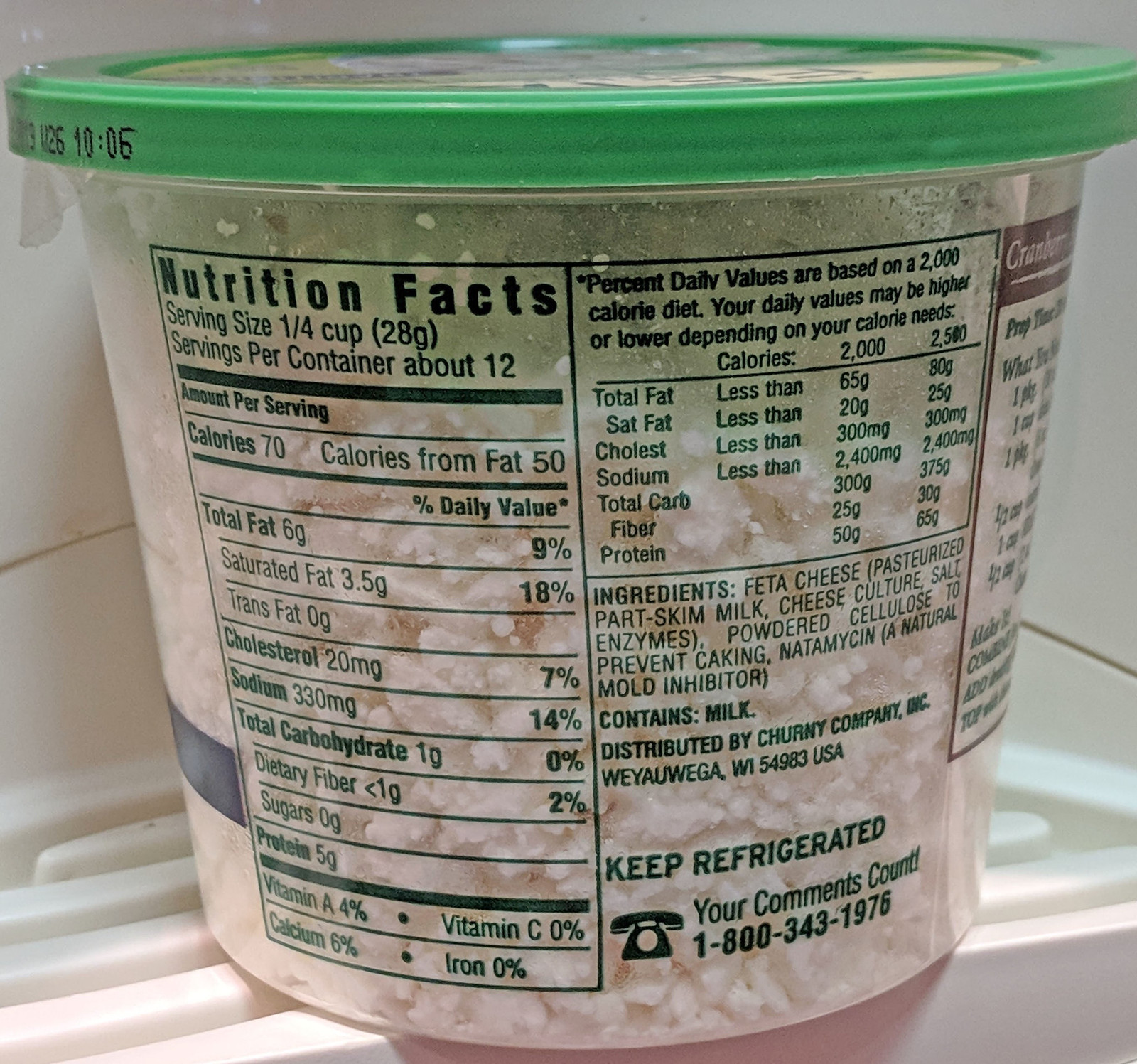A transparent plastic container with a green cap is prominently positioned inside a refrigerator, as suggested by the shelving and background elements. The container has an illegible yellow design or print on the lid. The front of the container features detailed nutrition facts in green print, while a green bar stripe is noticeable toward the bottom left. Near the bottom of the container, a small telephone icon accompanies the text "Your comments count" followed by the phone number "1-800-343-1976". Through the clear plastic, the contents of the container appear to be crumbled feta cheese.